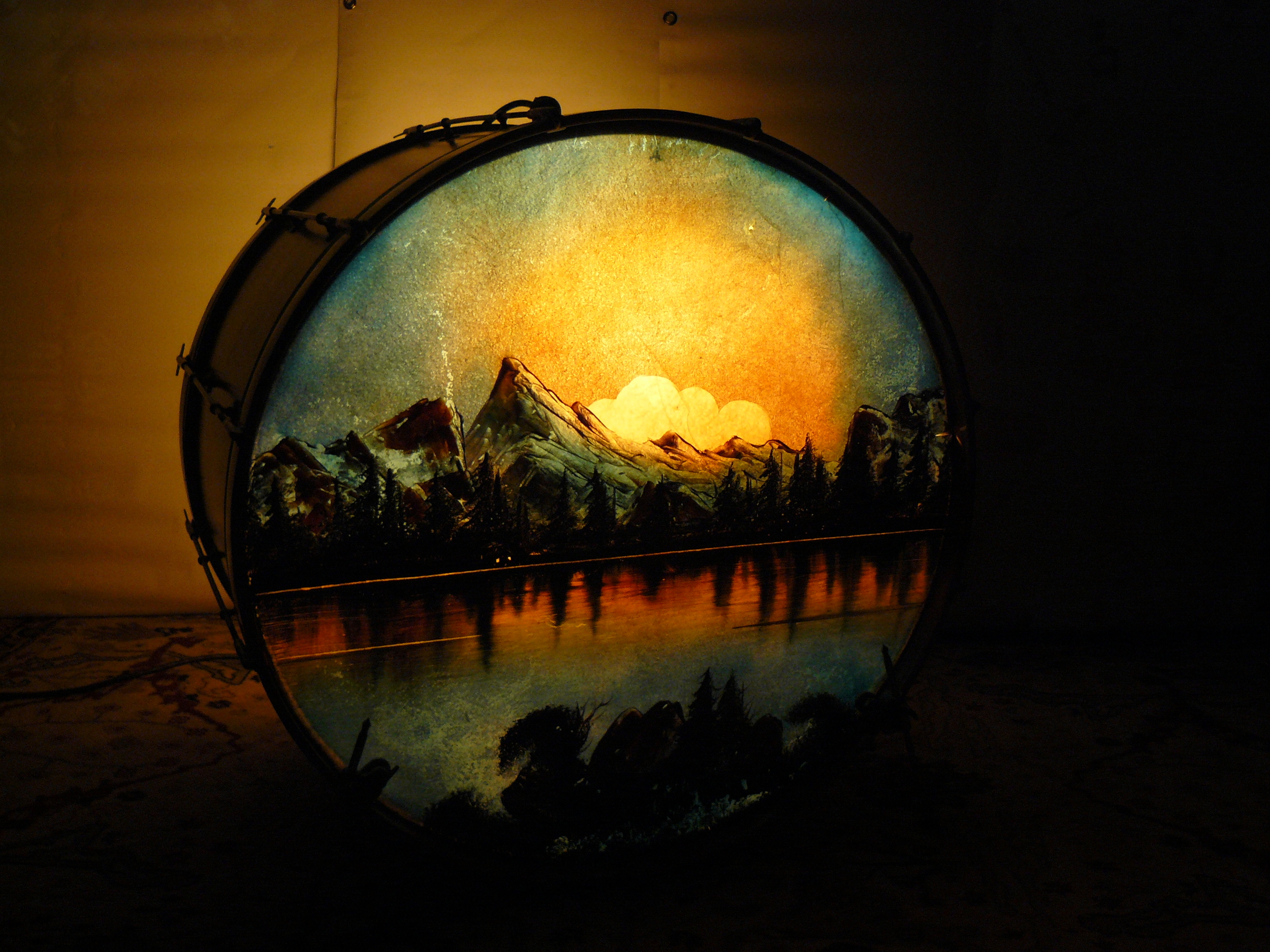This image features a detailed painting on a circular surface that resembles the end of a bass drum, set against a potentially soft, dark background that could be a tent wall or tarp. The overall color scheme is primarily dark browns and dark yellows, especially around the edges. The central focus of the painting is a landscape scene, featuring a sunrise or sunset with golden white clouds. At the apex of the scene is a bright circle of gold, fading into light blue, suggesting the transition of the sky. Below, rugged mountains are rendered in brown hues and are reflected in a serene body of water, along with the mirrored image of some trees. The drum-like surface also features unique textures and notches, adding to the antique feel of the piece. The landscape within the circle is meticulously detailed, creating an almost mirror image of the mountains and water, highlighted by the luminous backlighting which emphasizes the scene's rich colors and intricate details.